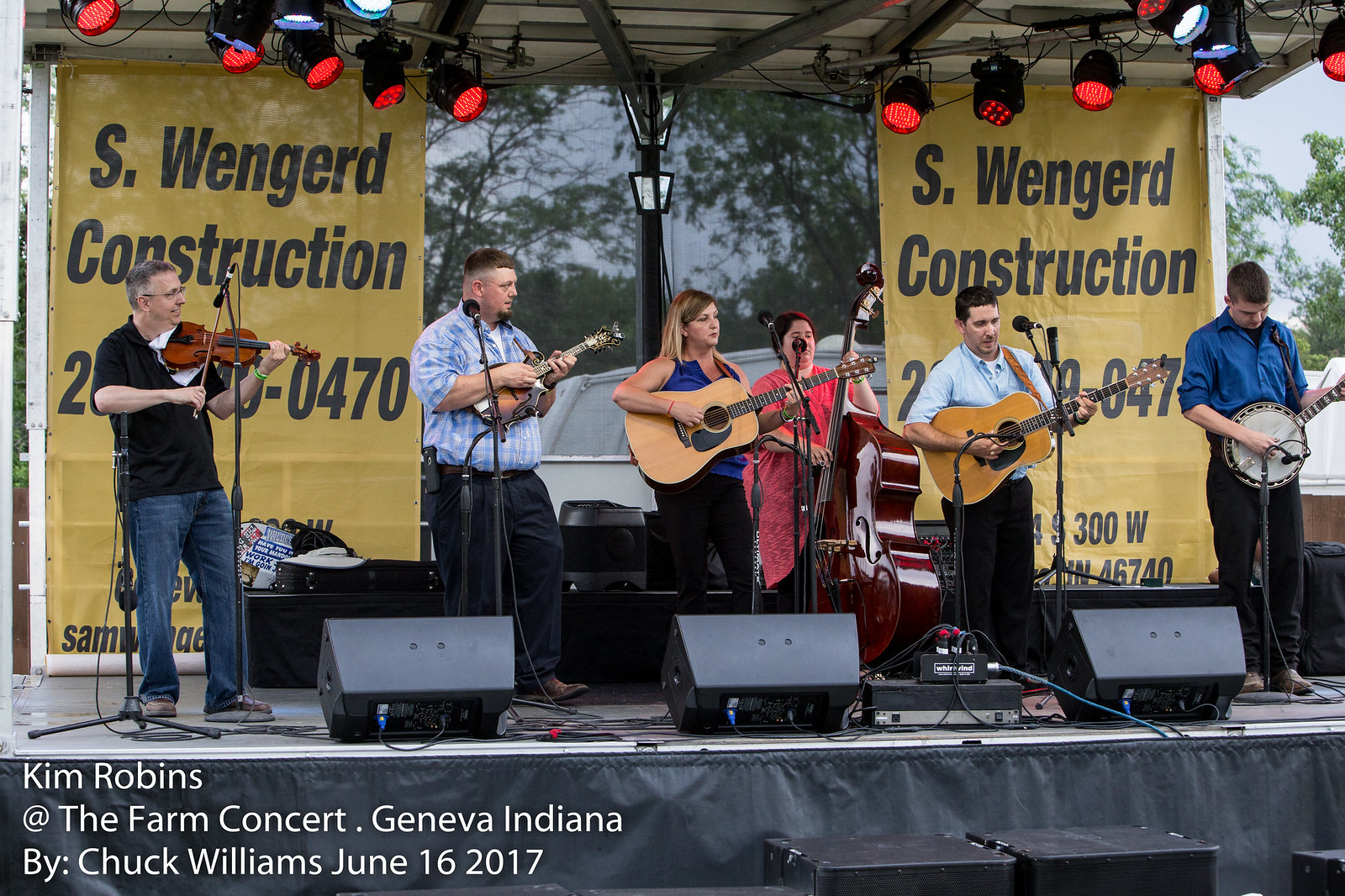The image captures a lively concert scene featuring a six-member band playing on an outdoor stage. Positioned from left to right, the ensemble includes a man playing a violin, a heavyset man holding a mandolin, a woman strumming an acoustic guitar, another woman playing an upright bass, a man with an acoustic guitar, and, at the far right, a man plucking a banjo. Each musician stands before a microphone, suggesting they are singing as well as playing their instruments. The stage is equipped with red spotlights above them, casting a warm hue in the dusk light. Behind the performers, two yellow banners display "S. Wengerd Construction" along with a phone number, indicating the event sponsor. Additional text overlay at the bottom of the photo reads, "Kim Robbins at the Farm Concert, Genova, Indiana, by Chuck Williams, June 16, 2017."